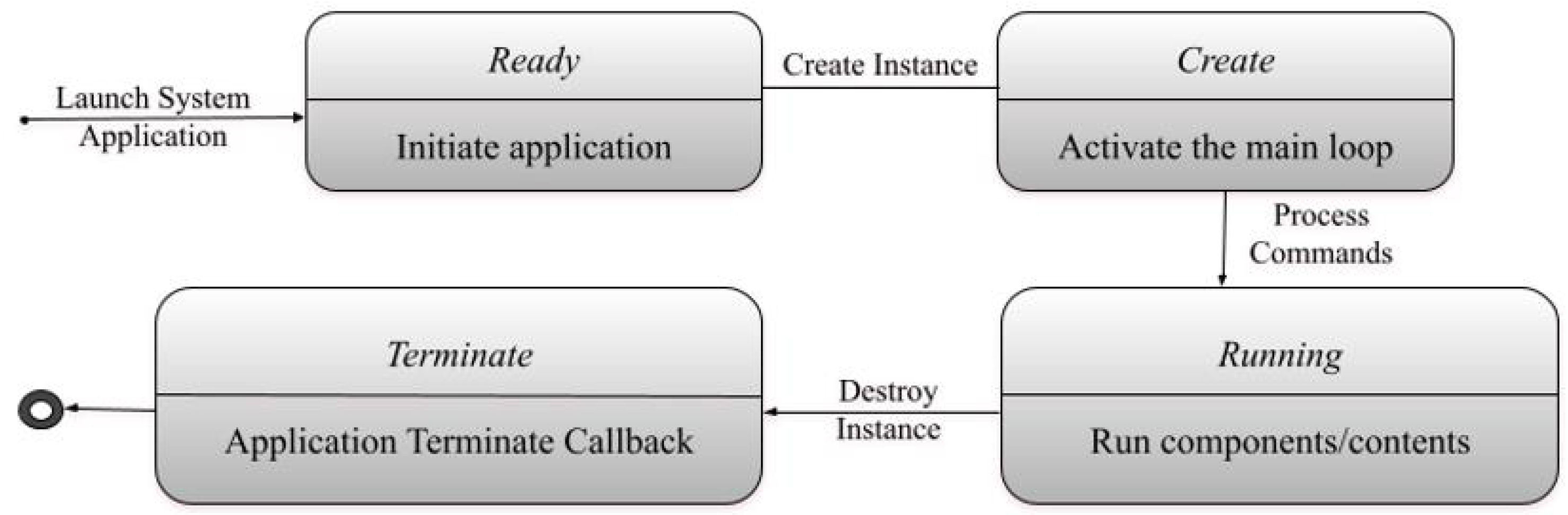The image is a detailed flowchart diagram representing the lifecycle of a system application, using black text on a white background with various shades of gray for the rectangles and lines. The flowchart begins with a command, "Launch System Application," leading to the first rectangle labeled "Ready" with "Initiate Application" underneath it. An arrow from this rectangle indicates the next step, "Create Instance," connected to the second rectangle labeled "Create" with "Activate the Main Loop" underneath. 

Following this, a downward arrow labeled "Process Commands" leads to a larger rectangle containing "Running" and "Run Components/Contents." From this larger rectangle, a right-to-left arrow labeled "Destroy Instance" points to another rectangle labeled "Terminate" with "Application Terminate Callback" underneath. The flowchart concludes with an arrow pointing to a black circle with a white center. The entire diagram is monochromatic with the only colors being black, white, and grayscale.